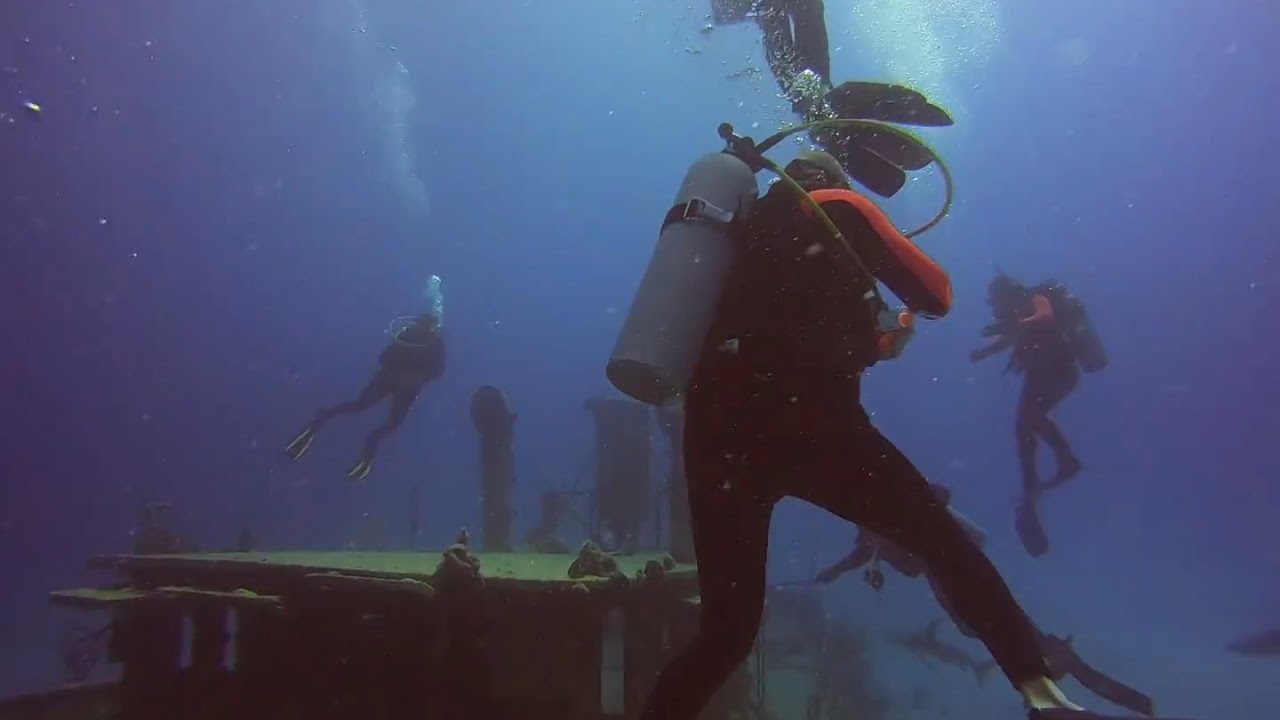In this horizontal rectangular underwater photo, the scene captures a group of scuba divers amidst a dark blue, almost purple, murky environment. In the foreground, a scuba diver dressed in a red and black wetsuit, with flippers on his feet, has his back to the camera. An air tank with a greenish compartment is strapped to his back, with a hose extending around to his front. He wears a mask that releases bubbles as he exhales. To the right, another diver is seen descending into the depths, while further in the background, more divers can be vaguely distinguished, all dressed in similar black wetsuits. The divers appear to be exploring a sunken structure, possibly a ship, hinted by the greenish element resembling felt-covered wood visible on the left side. Sunlight filters through the water, casting an ethereal glow, with the center of the image being brighter than the darker blue periphery. The formation and the sunken objects suggest an explorative dive, with the divers seemingly in a circular arrangement around the submerged area.